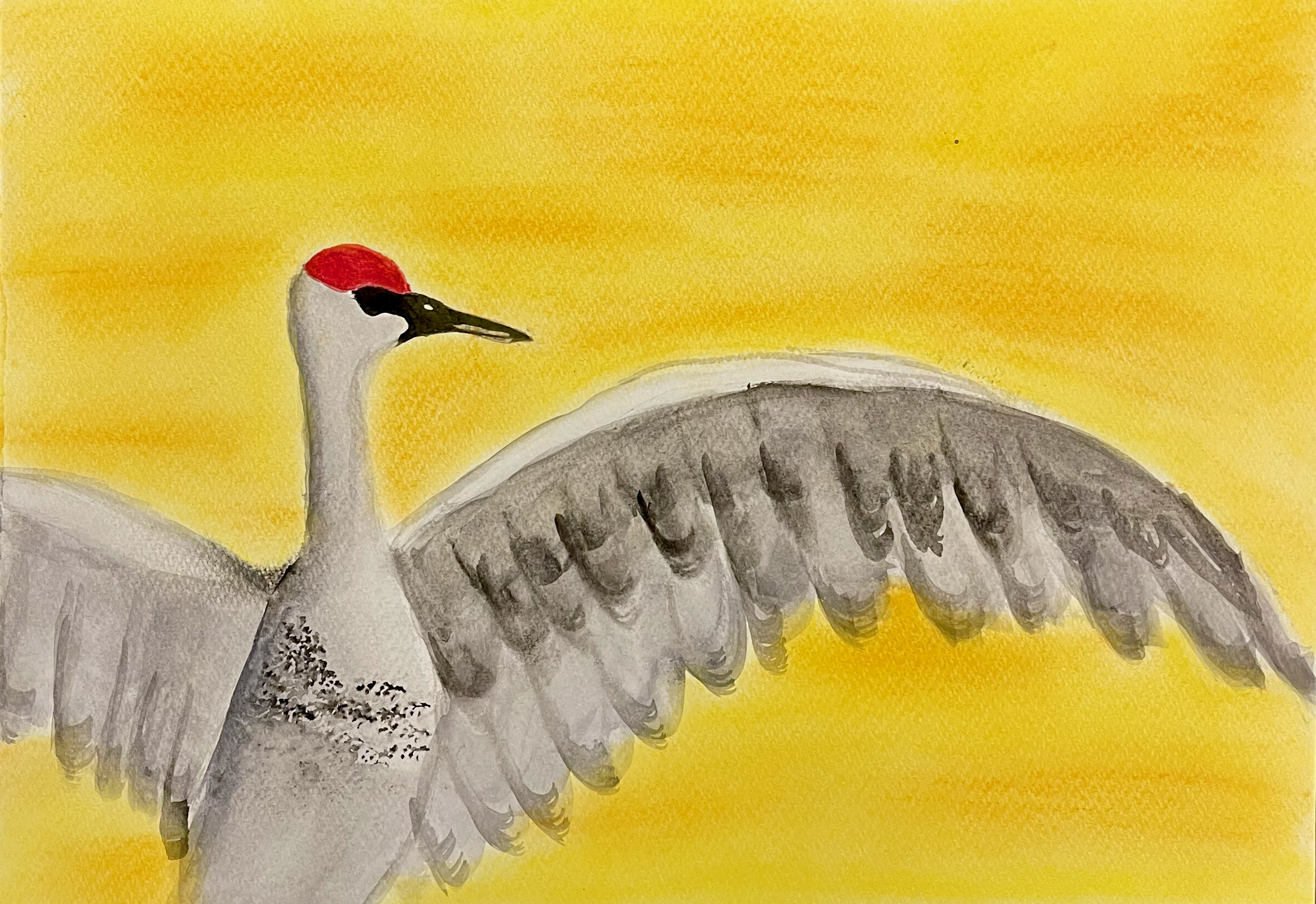The image depicts a detailed watercolor painting of a large bird, likely a sandhill crane, set against a vibrant yellow background, hinting at daylight, possibly during sunrise or sunset. The bird dominates the composition, showing primarily its chest, torso, head, and an extended wing, while the other wing is partially cut off by the painting's frame. The crane is predominantly white with grey shadings on its wings and the bottom of its neck, along with specks of black on its chest. Its head is distinctively red, and it features striking black eyes and a long, narrow, pointed black beak. The painting skillfully blends various shades of yellow in the background, adding depth and texture, enhanced by the visible canvas underneath. The bird's posture suggests it is either standing or in mid-flight, with its neck extended and its wings partially spread, creating a dynamic and elegant portrayal of wildlife artistry.